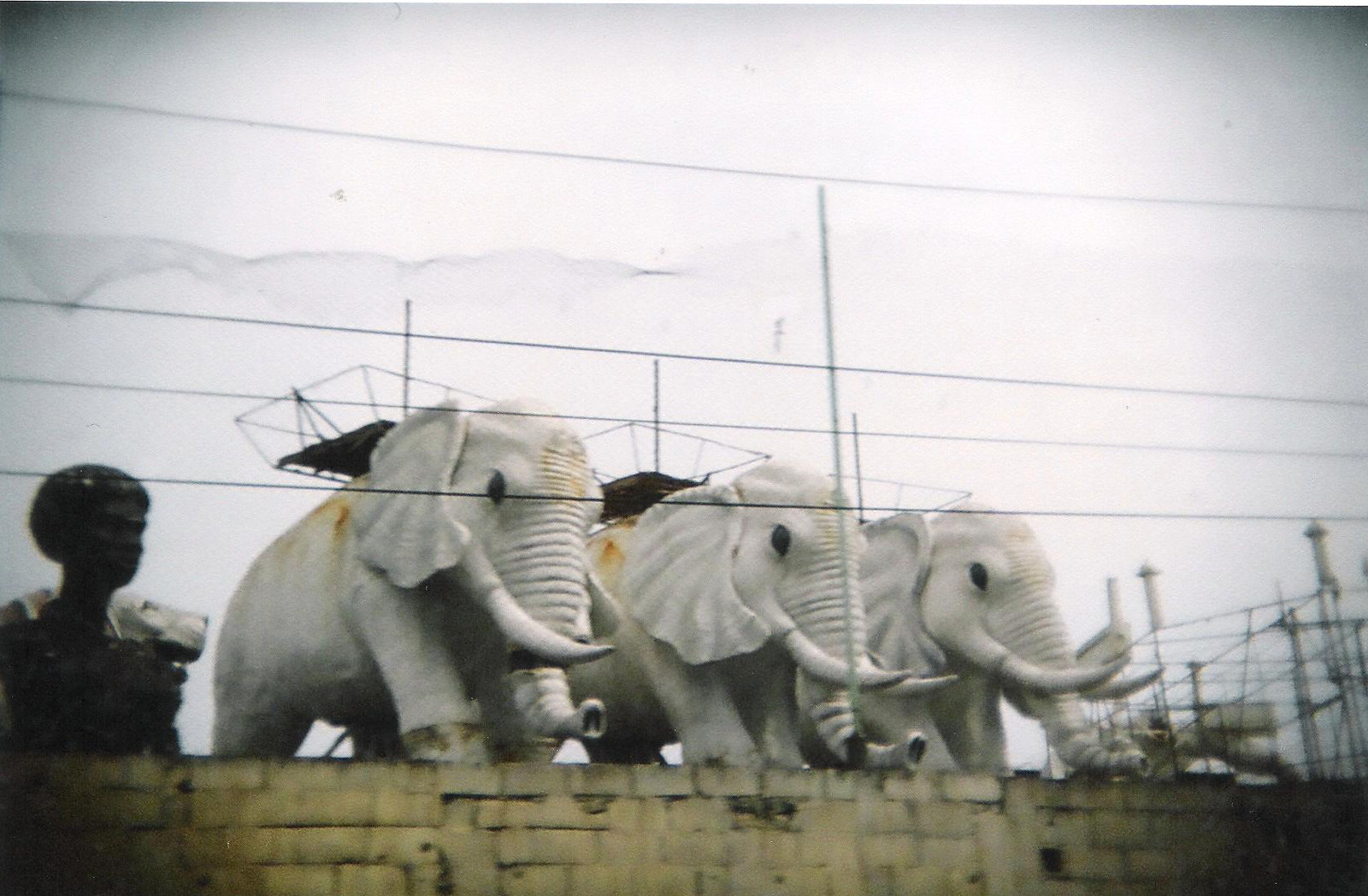The image is a slightly blurred photograph featuring three large, statue-like African elephants, primarily whitish in color with patches of rust in hues of yellow, orange, and brown. These elephants are positioned centrally and appear to be made of ceramic. They are adorned with structures resembling seats or derricks on their backs, possibly for carrying passengers, with their feet placed against or atop a beige-colored brick wall that is painted white at the bottom. To the left of the elephants stands a figure of a person with dark skin, likely a model rather than an actual person, adding to the lifelike quality of the scene. The backdrop includes a pale wall and a complex wire structure resembling cages or roller coaster elements on the right side. The overall photograph has a vignette effect, with darker edges and a predominantly grey, muted palette, giving it a slightly monochromatic and staged appearance. The sky above is grey, enhancing the subdued lighting that appears non-natural, accentuating the central figures.